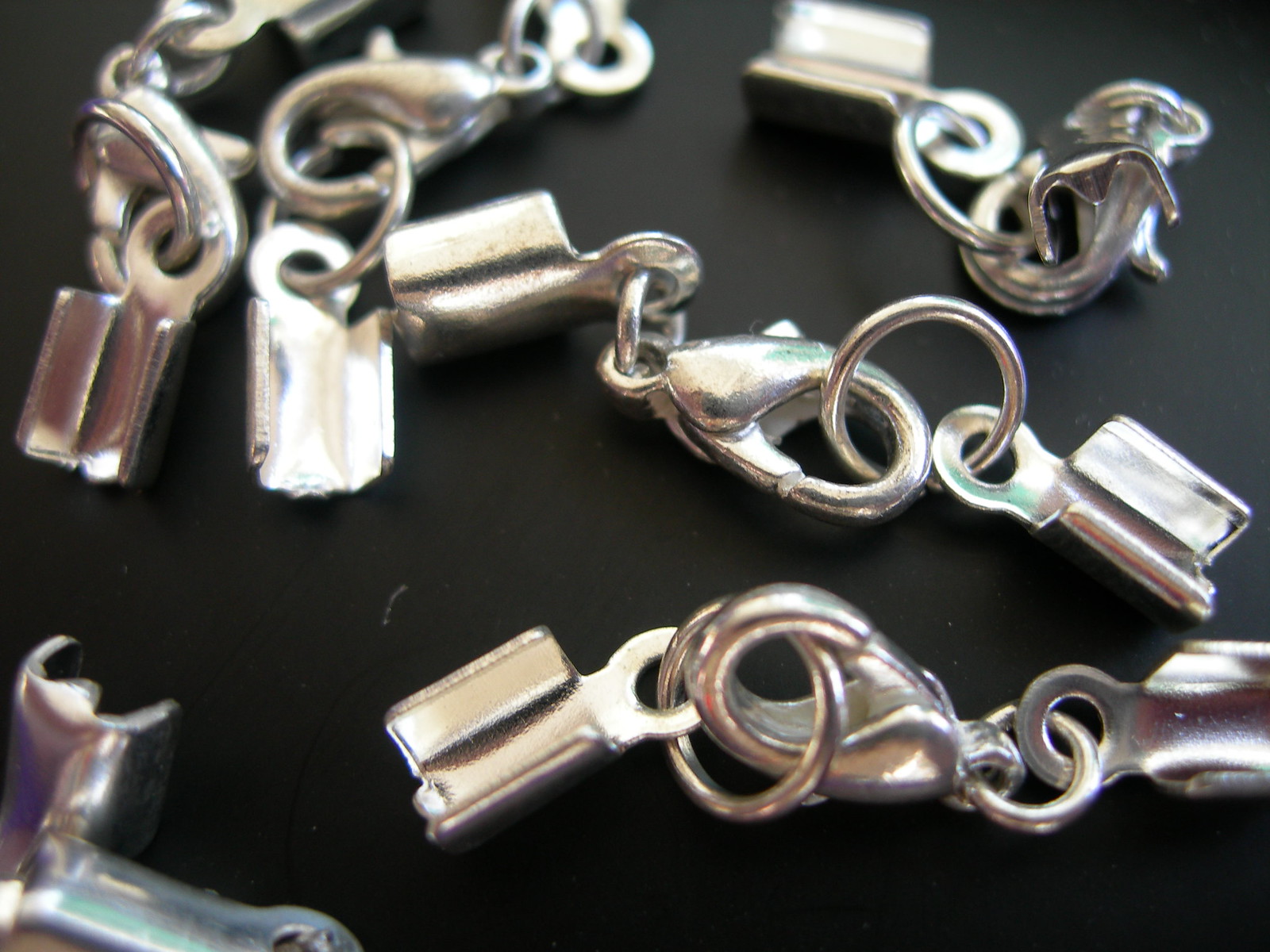The image displays a silver-colored linked chain, possibly from a broken necklace or bracelet, sprawled across a black, shiny surface that could be a table or countertop. The chain comprises several identical pieces, each no longer than two inches, repetitively structured with connecting round and square-shaped components. These components include small circles, some looping once and others twice, connected by metal clasps that could potentially be used to secure the chain. The meticulously organized segments, consisting of seven linked pieces, add a repetitive yet intricate design to the chain, which is devoid of any written text or noticeable inscriptions.